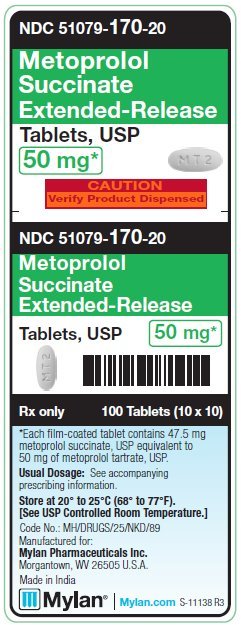The image is a screenshot of a phone displaying an advertisement for medication. The screen features a light blue border encompassing the content. At the top, a black bar presents "NCD," followed by a series of numbers separated by hyphens. Below that is a green bar with the text "Metoprolol Succinate Extended Release." The words "Tablets, USP, 50 mg" are in white, accompanied by an asterisk and enclosed in a green circle.

The advertisement includes an image of the tablet for reference. Below the green section, an orange and burgundy caution message reads "Caution: Verify Product Dispensed," which is repeated underneath. Adjacent to this warning is a barcode, indicating that the product can be scanned, commonly used in prescription verification.

Further down, the text specifies, "RX only," "Prescription Only," and details the quantity as "100 tablets (10x10)." Additional information in light blue mentions that each film-coated tablet contains 47.5 mg of the active drug, USP, equivalent to 50 mg as advertised. The usual dosage instructions, storage guidelines, and the note that the product is manufactured by Mylan in India are also included. Overall, the ad appears cluttered and somewhat suspicious, raising concerns about its trustworthiness.